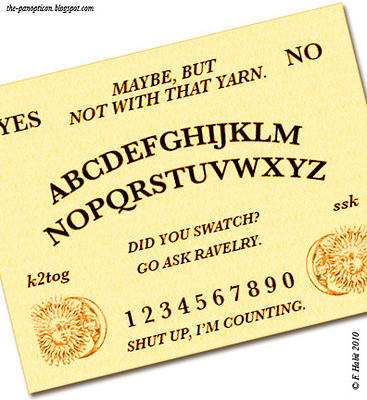The image depicts a cropped photograph of a whimsical, non-traditional Ouija board featured on a webpage. The board's background is a light tan, resembling plywood or solid paper, with detailed etchings and humorous text. In the upper left corner is the word "Yes," and in the upper right, "No," with "Maybe, but not with that yarn" centrally positioned between them. Below this, the board displays the entire alphabet in two lines, followed by a line of numbers from one to nine and zero. In the lower section, a quirky phrase reads, "Did you swatch? Go Ravelry," and further down, "Shut up, I'm counting." The board is adorned with sun and crescent moon logos on both the lower left and right corners, adding to its playful and satirical design. The upper left corner of the photograph includes a partial text indicating a blog or webpage, hinting at its online origin.